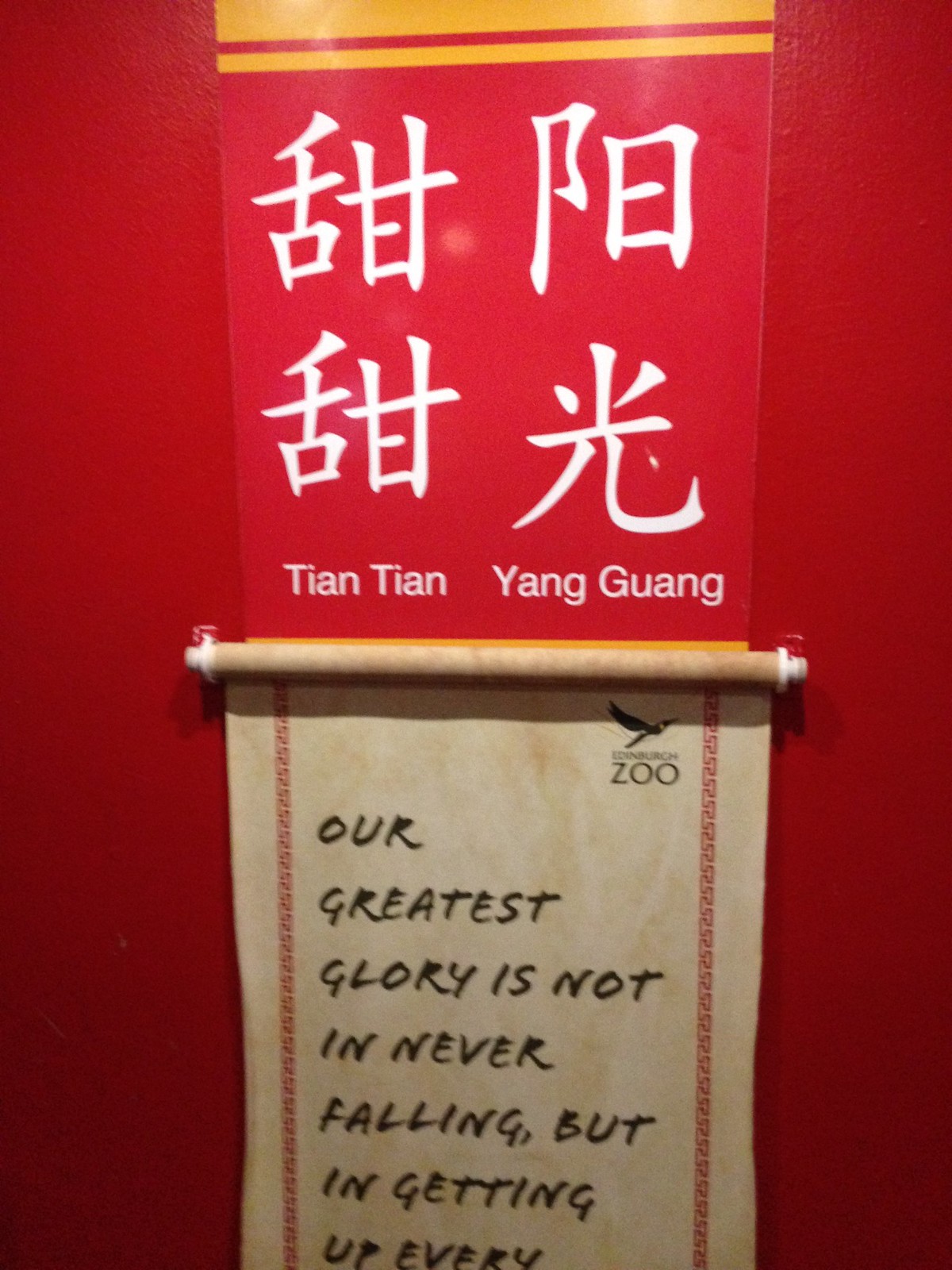The photograph depicts a visually striking scene featuring a poster against a deep red background. At the top middle of the horizontal image are two yellow horizontal lines extending vertically for about a third of the image's height. Below these lines is a lacquered red rectangular surface adorned with white Chinese characters. These characters form a loose rectangle, with the top and bottom left characters being identical, as well as the top and bottom right ones. In the center of this arrangement, in smaller white letters, it reads "Tian Tian" with both Ts capitalized. To the right, in similar white letters, it says "Yang Guang," with the Y and the G capitalized.

Beneath the lacquered sign hangs an antique-looking scroll, with its edges slightly worn and resembling old-fashioned, possibly burnt or indented paper. An eagle or bird is stamped in black ink at the top of the scroll, which also features black calligraphic text that reads: "Our greatest glory is not in never falling, but in getting up every..." The text cuts off, leaving the final word unreadable. Around the scroll are delicate vertical lines patterned in a lacy, filigree style, adding an ornate touch.

This combination of striking red hues, traditional Chinese characters, and inspirational English text suggests the poster may be aimed at both Chinese and international audiences, possibly in a tourist area or as a piece of vintage signage dating back several decades.